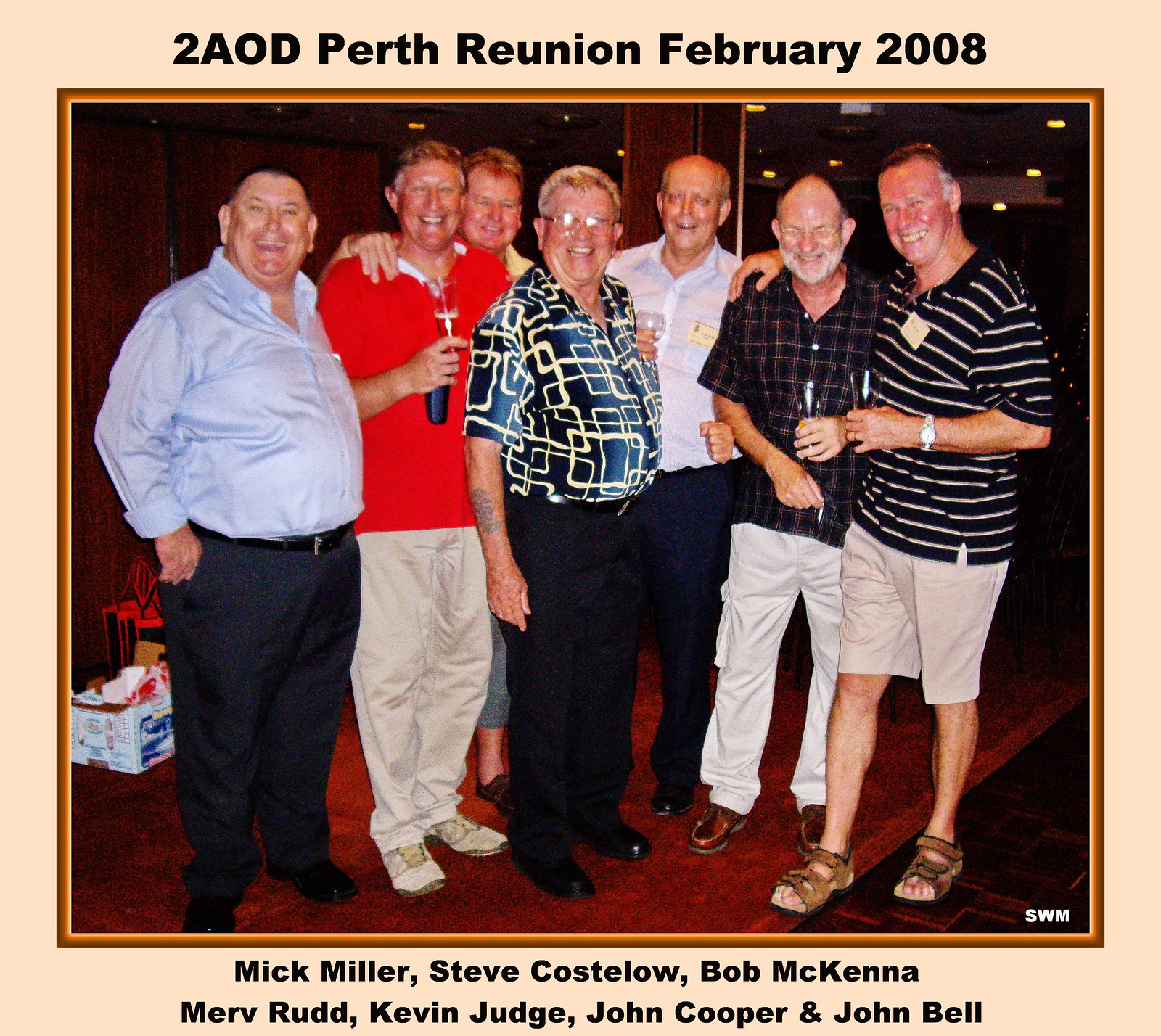In this photograph, titled "To AOD, Perth Reunion, February 2008," seven older gentlemen are casually dressed and gathered for a reunion, most likely commemorating their time together in the military. The image has a gold-like border with black text at the top and bottom. The men are identified in black print at the bottom as Mick Miller, Steve Costolo, Bob McKenna, Merv Rudd, Kevin Judge, John Cooper, and John Bell. From left to right, Mick Miller, a larger gentleman in a light blue shirt and navy pants, stands next to Steve Costolo in a red shirt and beige khakis. Behind Steve, only the head of Bob McKenna with glasses is visible. In the center, Merv Rudd, another larger man, wears a blue shirt with a yellow pattern and black slacks. To his right, Kevin Judge, in a white shirt, stands next to John Cooper in a black striped shirt and white pants. John Bell, on the far right, wears a black t-shirt with yellow horizontal stripes and beige pants. The setting, possibly a hotel or restaurant, and the casual attire, suggest a relaxed and enjoyable reunion, with many of the men holding drinks.